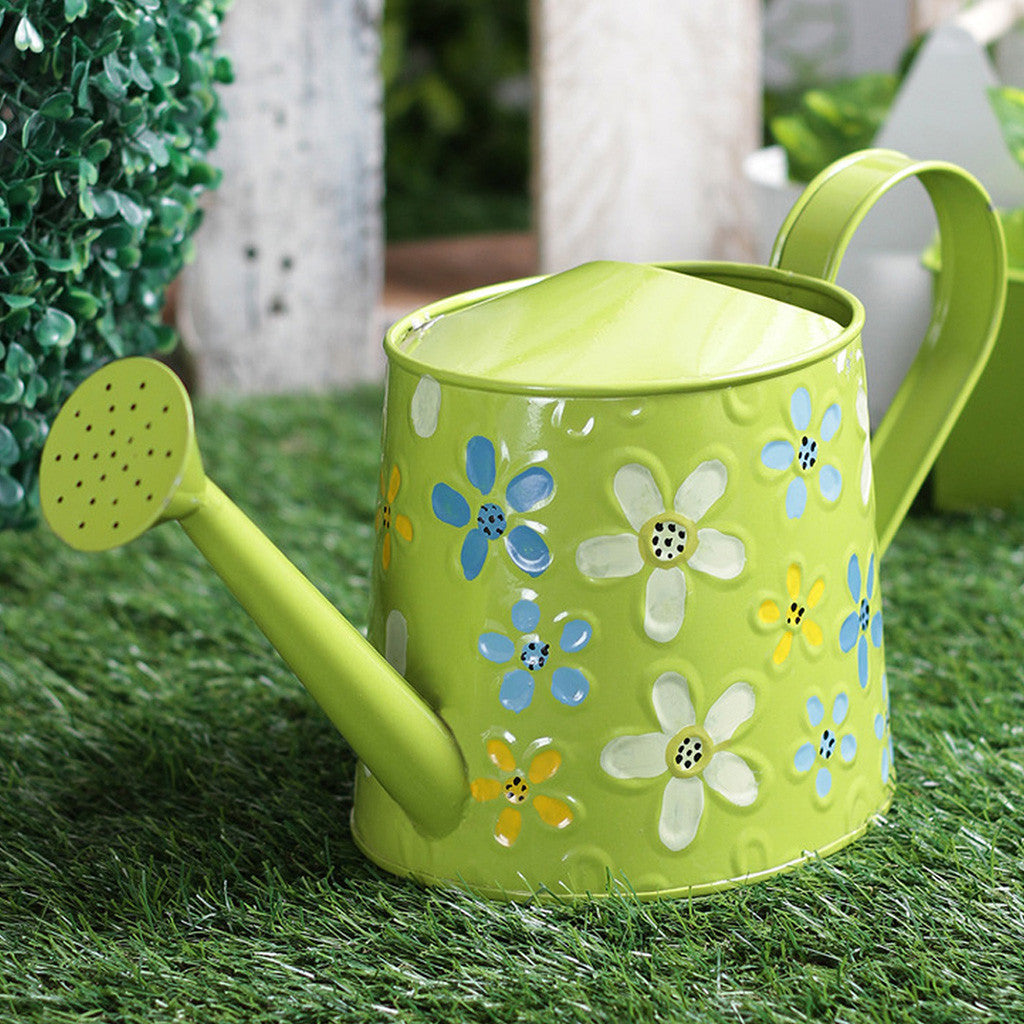This close-up outdoor photograph features a light greenish-yellow metal watering can, positioned on a lush, green grass. The can is adorned with simple, daisy-shaped flowers painted in white, blue, dark yellow, and black. Its spout, which is to the left and ends in a perforated, shower head-like nozzle, is slightly tilted forward. The handle, positioned to the right and higher than the body of the can, forms an arcing loop. The blurred background showcases green vegetation and a hint of a white picket fence composed of two white boards. To the left of the can, a lush green bush partially enters the frame, adding to the natural setting. This charming image, potentially suitable for promotional use, captures the essence of gardening with its vibrant colors and inviting outdoor scene.